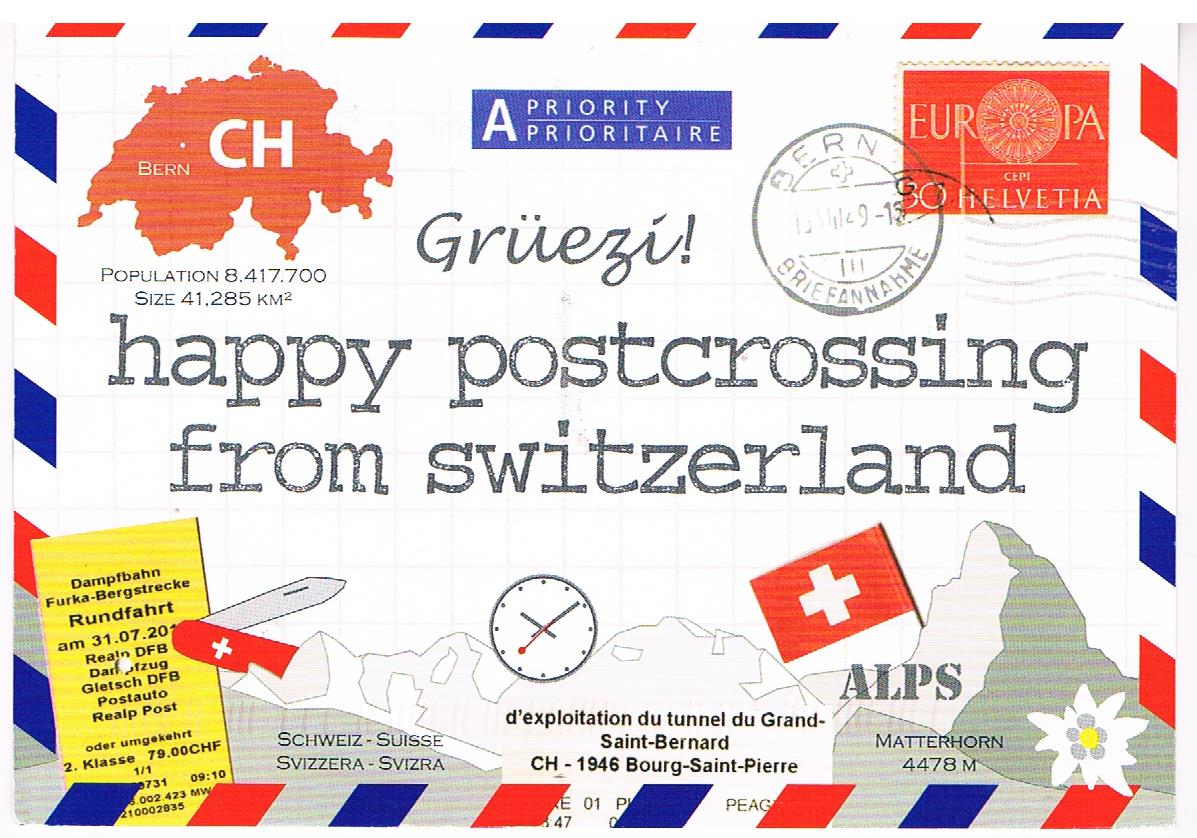The image is a detailed postcard designed with a striking red, white, and blue border. At the top, in cursive, it reads "Grüezi!" with an exclamation mark, a Swiss greeting. Dominating the center is the message "Happy Post Crossing from Switzerland" written in faded black text. Below it, there is a blue rectangular banner displaying "Priority" and "Prioritaire." The postcard features various Swiss iconic symbols around its edges: a small map of Switzerland marked with "BERN" and the country code "CH" in the upper-left corner; an image of the Swiss flag, red with a white cross, positioned prominently. Additionally, there are sketches of a Swiss army knife and a clock emblematic of Switzerland's timekeeping legacy. There's a stamped mark from the post office in black ink on the right side. The bottom left corner showcases a yellow banner with Swiss terminology, and nearby, a picture of the Alps mountain range. The postcard is set against a clean, white background, making these details stand out vividly.